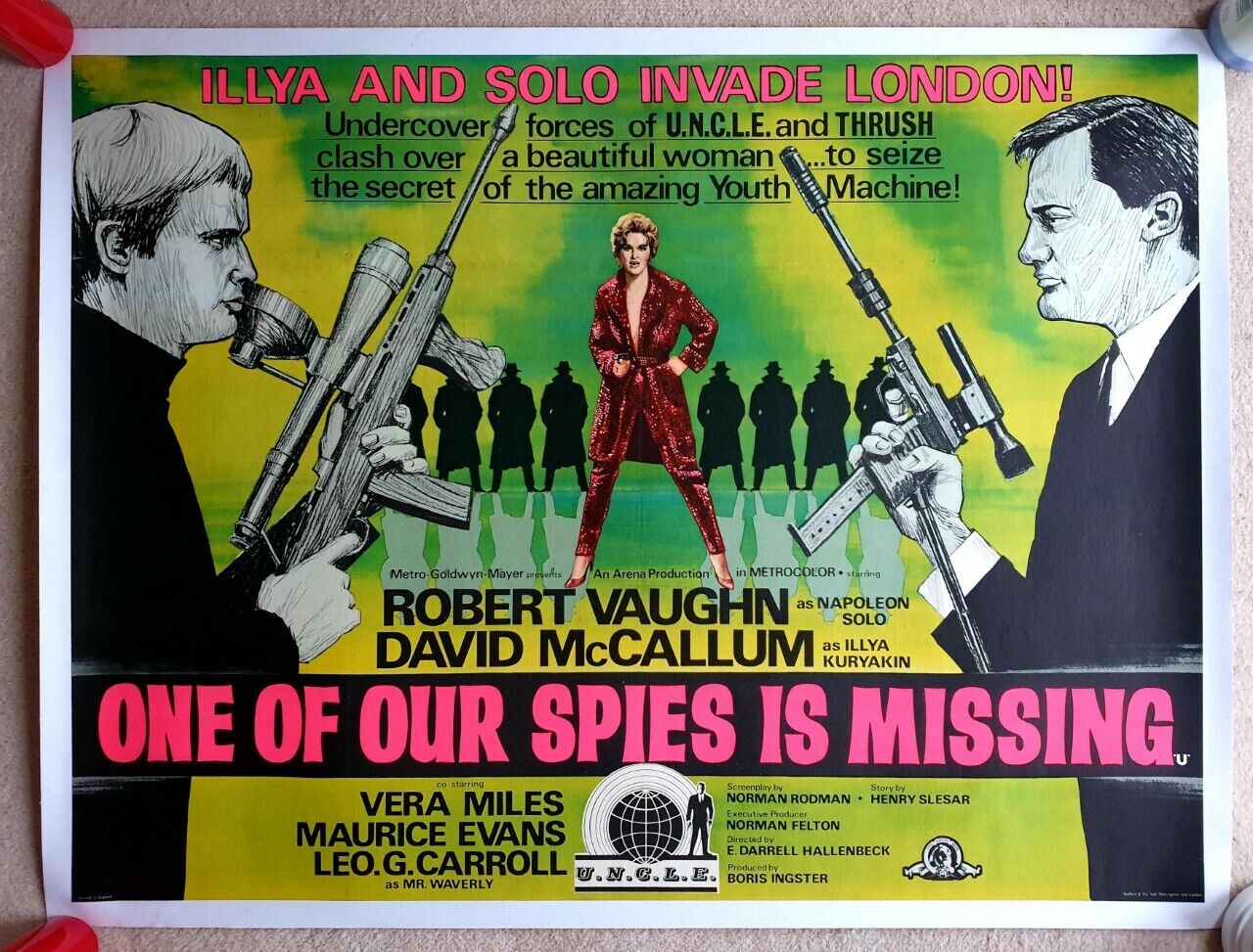This image is a horizontally oriented, vintage movie poster pinned at the corners to a billboard or bulletin wall. The headline at the top reads, "Ilya and Solo Invade London. Undercover forces of UNCLE and Thrush clash over a beautiful woman to seize the secret of the amazing youth machine." Dominating the center of the poster is a woman in a striking red sequined jacket and pants, paired with red high heels. She holds a pistol, exuding a sense of danger and allure. Flanking her are two illustrated men on the left and right, each gripping a gun and facing one another, underscoring the tension between them. The color palette includes vibrant hues of tan, red, white, pink, green, yellow, black, and different shades of gray and maroon. The bottom of the poster features the title in prominent pink text: "One of Our Spies is Missing." This intricate blend of characters and vivid colors suggests an action-packed, espionage narrative central to the storyline.